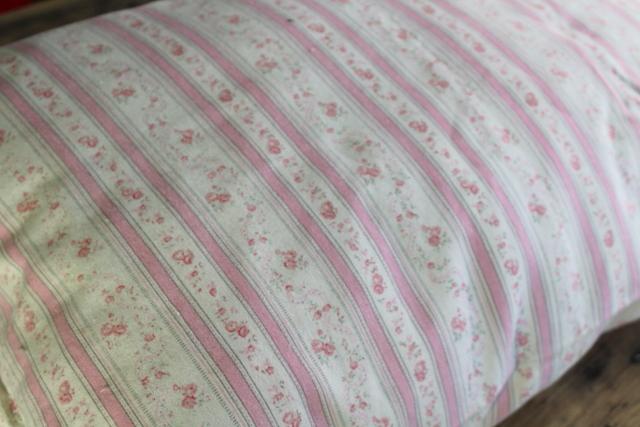The image features a fluffy white pillow adorned with a repeating pattern. The design begins with thin vertical gray lines, followed by thick pink stripes, and then a column of delicate pink flowers. This sequence continues across the pillow. The fabric appears slightly blurry and faded, especially towards the top right. The pillow, which is placed on a brown surface, is oriented such that its width is longer than its height. The overall aesthetic includes subtle baby pink colors and intricate floral details, creating a soft, inviting look.